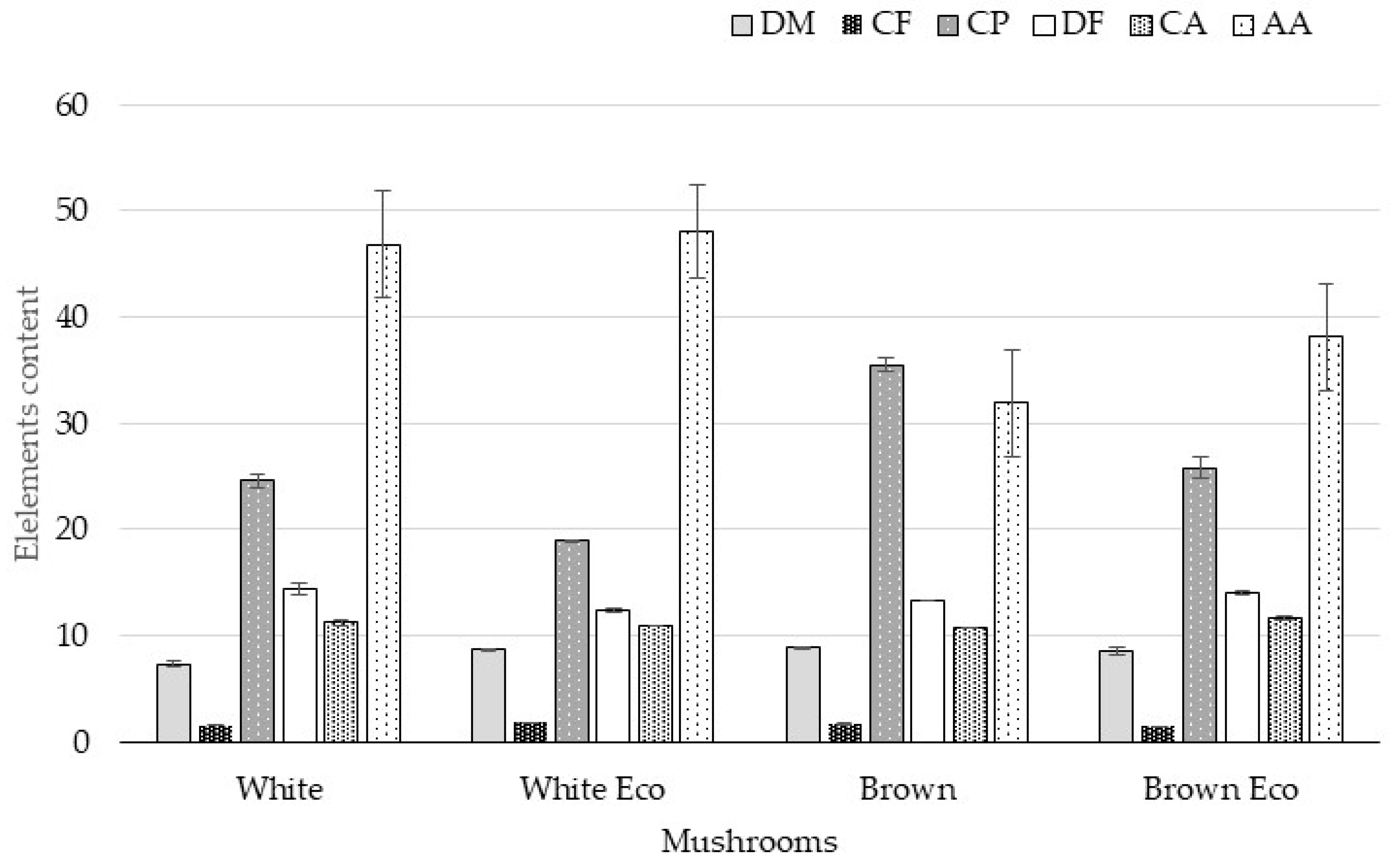The image is a detailed black and white bar graph illustrating element content based on different mushroom categories. On the left side, the y-axis is labeled "Element Content" and ranges from 0 to 60 in intervals of 10. The x-axis at the bottom specifies mushroom types: White, White Eco, Brown, and Brown Eco. Each category features six bars, corresponding to a legend at the top that indicates varying shading or patterns for the following labels: DM, CF, CP, DF, CA, and AA. The highest element content is observed in AA across most categories, whereas CF consistently shows the lowest levels.